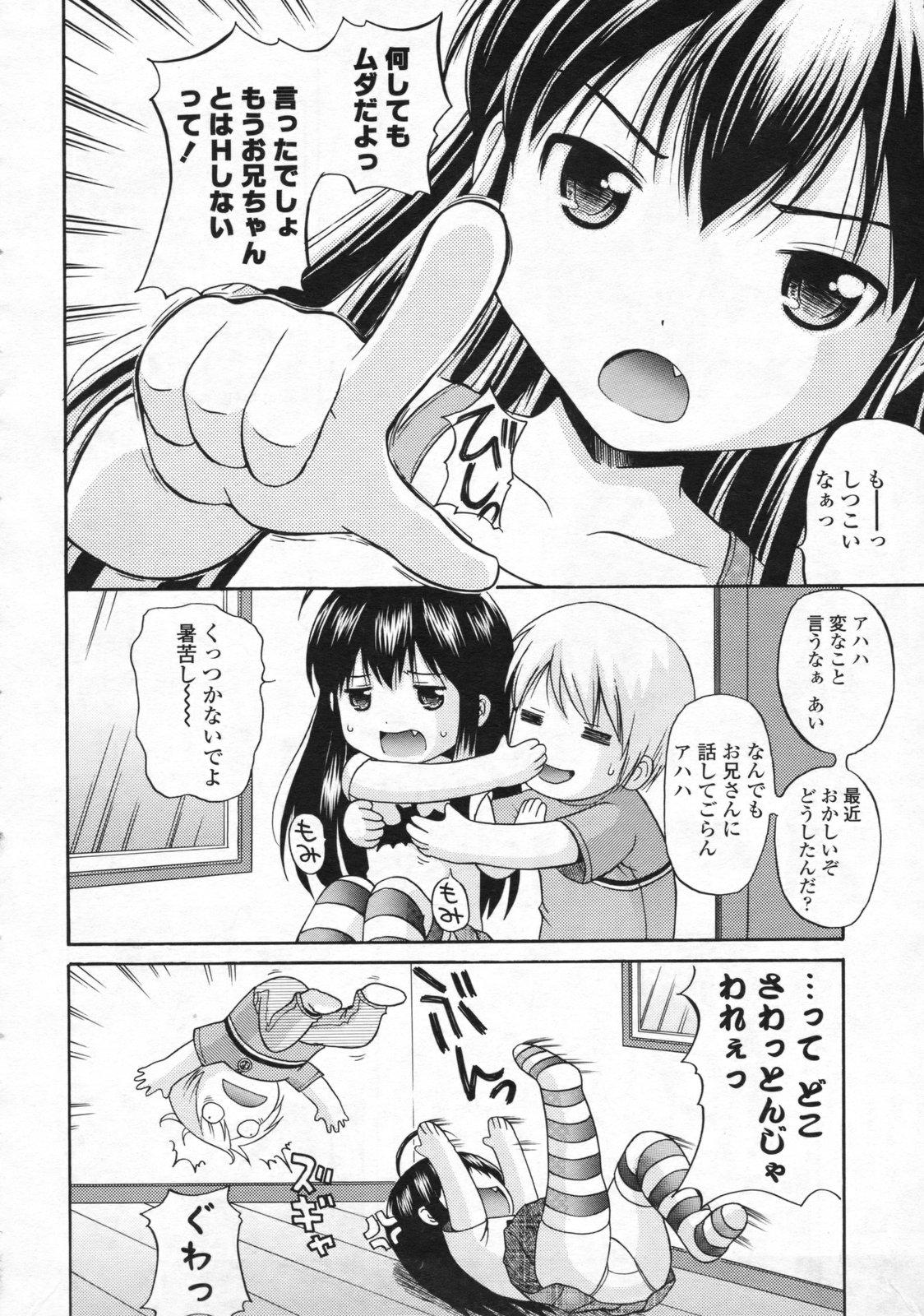In this black-and-white three-panel vertical manga comic strip, the top and largest panel showcases a young Japanese girl with long black hair and heavy bangs pointing her finger and angrily screaming, with several word bubbles in Japanese around her. The middle, smaller panel features the same girl with tears in her eyes hugging a boy with blonde hair, who is wearing a gray top and appears to be laughing. The final panel, the same size as the middle one, depicts the girl lying on her back while playfully flipping the boy, who has wide, shocked eyes, into the air with her feet. The boy appears to be doing a somersault backward, his arms extended as he is about to hit the floor. Vertical Japanese script panels are present in both the middle and final panels, providing their dialogue.